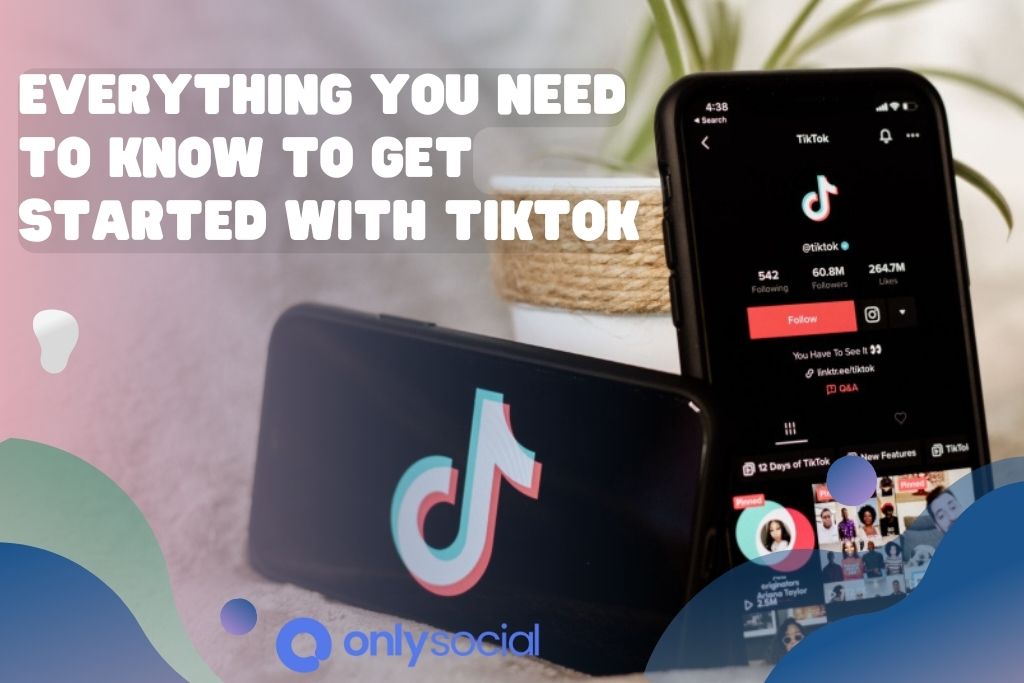The image features a purplish-gray background adorned with abstract gray and blue lines swirling at the bottom without any distinct pattern. Scattered across the left side are small white globs that seem to float weightlessly. At the bottom, there is a prominent blue circle with a gray center, accompanied by the text "Only Social" in white and black. In bold, white capital letters, the text "EVERYTHING YOU NEED TO KNOW TO GET STARTED WITH TIKTOK" is prominently displayed. 

Two smartphones are depicted: the one on the left showcases the TikTok logo, while the phone on the right displays the TikTok home page, complete with follower counts, likes, and other interface elements. Below this, a red button is visible, and beneath it is a collage of photos featuring various TikTok users.